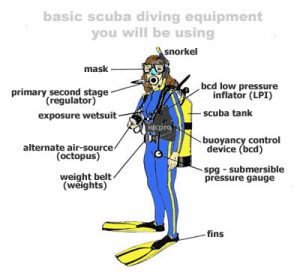The instructional image titled "Basic Scuba Diving Equipment You Will Use" depicts a detailed front-facing illustration of a person, likely a woman with light brown or dark blonde hair, suited up in bright blue exposure wetsuit with distinctive yellow stripes running along the arms and legs. She is equipped with essential scuba gear, which is meticulously labeled. The list begins with the snorkel and full mask, followed by the primary second stage regulator over her mouth, and the alternate air source, known as the octopus. Around her waist, she wears a weight belt and an SPG, or submersible pressure gauge. Her feet are fitted with yellow and black swim fins. On her back, a yellow scuba tank is strapped securely along with a buoyancy control device (BCD) that is connected to a BCD pressure inflator or low-pressure inflator (LPI). Each piece of equipment is marked with lines connecting to their respective labels, ensuring clear identification and understanding of their use for scuba diving training purposes.